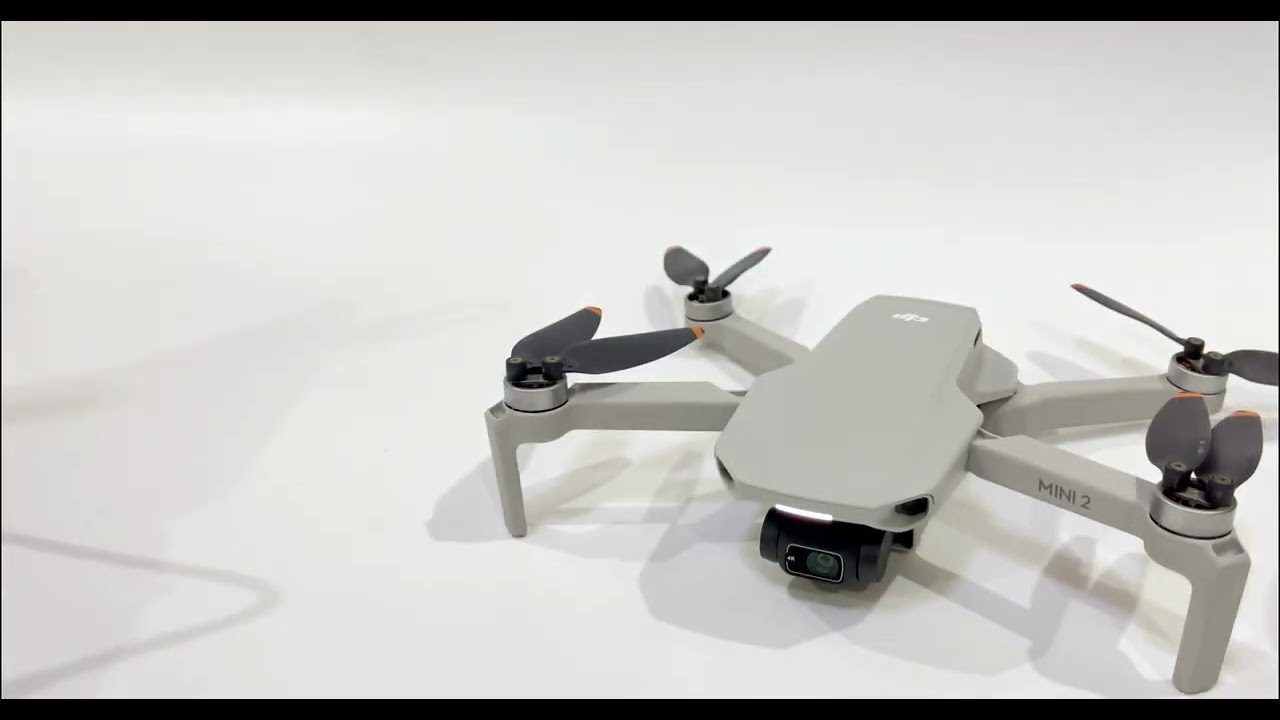The image depicts a Mini 2 drone positioned in the lower right quadrant against a white background. The drone, primarily light grey, features four arms each with black propellers that have small orange or copper tips. Notably, the left front arm is labeled with "MINI2." Below the central fuselage, which is also grey, a black camera lens or control area is visible. The drone casts a prominent shadow to the lower left corner of the image. Additionally, the image itself has black borders at the top and bottom edges.